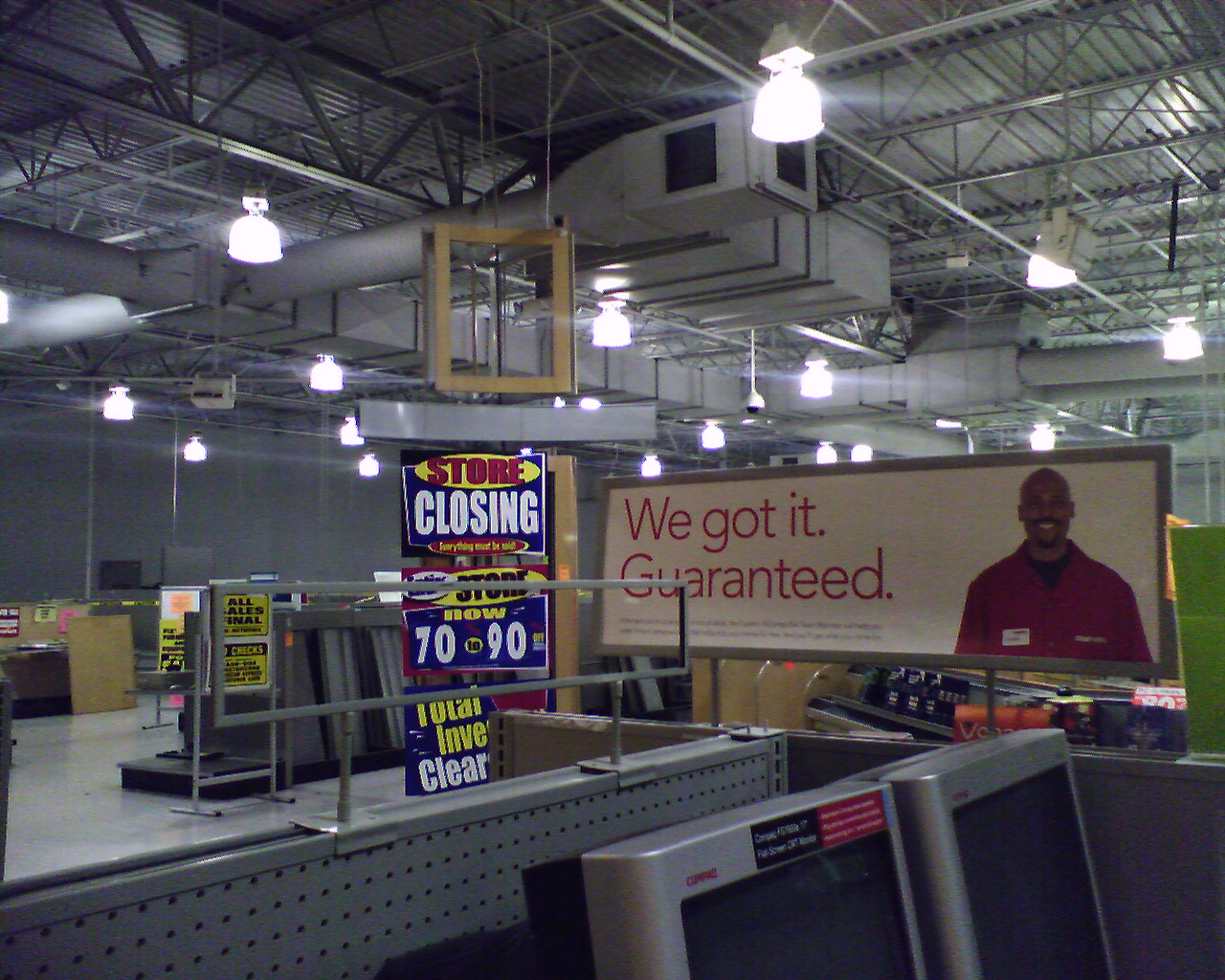The photograph captures the interior of a Staples store in its final days of operation. The store is well-lit with bright, white lighting emanating from the steel-barred ceiling. Various “Store Closing” signs, advertising massive discounts ranging from 70% to 90% off, are prominently displayed. The store sits mostly vacant, with numerous empty shelves and racks scattered throughout the space.

In the background, a cluster of older Compaq computer monitors is visible, hinting at the lingering inventory. A large, bold sign proclaiming “We Got It Guaranteed” hangs conspicuously, a poignant reminder of the store’s more bustling days. A lone employee, dressed in a red polo shirt and sporting a white name tag, stands amidst the hollowed-out aisles. The scene evokes a sense of desolation, as the near-empty store now resembles a vast warehouse due to its sheer emptiness.